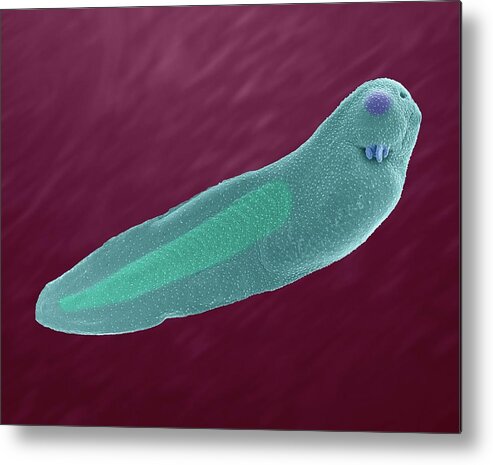The image features a maroon background with subtle textural details and shades of white. At the center, there is a peculiar sea creature, which appears somewhat like a thick, worm-shaped, cartoonish otter. This creature has a long, carrot-like body with fin-like arms on either side. The creature is predominantly greenish-gray with a lighter cone-shaped section inside, revealing a somewhat translucent organ. Its face, turned toward the viewer, showcases a purple nose, three to four prominent white buck teeth, and a single visible black eye resembling a small black hole. The image overall feels like it is inspired by a dot art style, leaving it uncertain whether it is hand-drawn, computer-generated, or painted. The entire scene has been encapsulated in a small, square format, giving it a portrait-like appearance that one might expect to see framed on a wall. It’s a distinctive art piece with a bizarre yet intriguing subject.